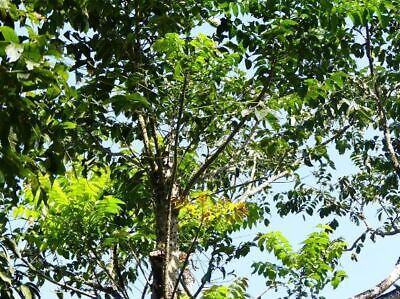The image showcases a vibrant, towering tree against a clear blue sky, captured from a unique perspective looking up from the base through the dense foliage. The prominent, sprawling branches are dotted with a variety of leaves that range from light to dark green, suggesting it is either spring or summer. Notably, there is a pruned limb, which adds an interesting detail to the tree's structure. On the lower portion of the image, there appears to be a white animal, possibly a squirrel, adding a touch of life to the scene. The leaves vary in size with larger ones on the left and smaller leaves towards the bottom, emphasizing the rich diversity within this captivating natural snapshot.